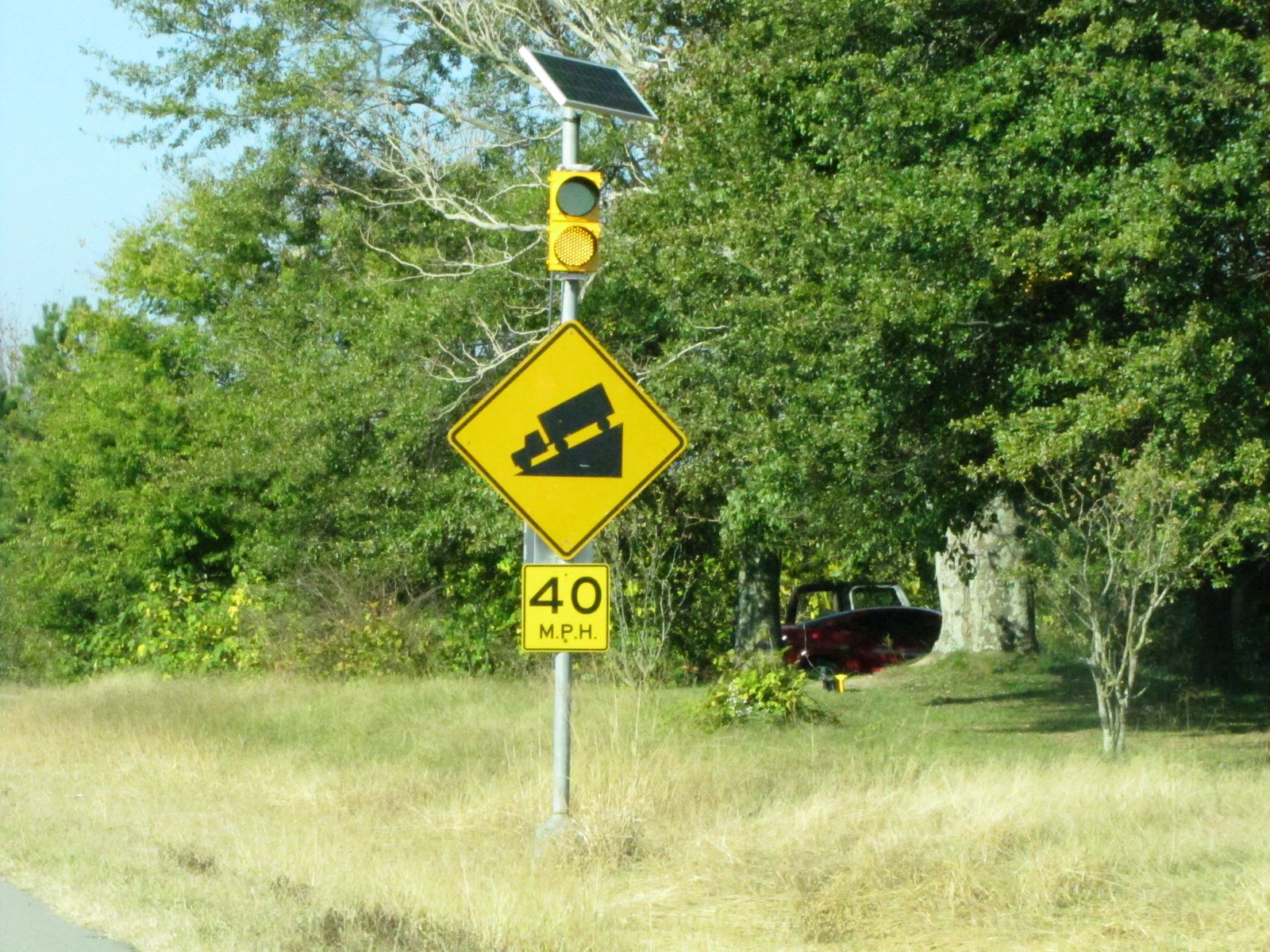On a sunny day, the image captures a prominently positioned traffic warning sign. The diamond-shaped, yellow sign features a black truck icon descending an incline, signaling a steep downward slope. Below the icon, text reads "40 MPH," indicating a speed limit of 40 miles per hour for vehicles on the incline. The sign is mounted on a silver pole, which also hosts a solar panel at the top and a traffic light that likely switches between green and yellow.

The sign sits by a roadside lined with grass, which appears to be in poor condition, showing patches of brown among the dying blades. Surrounding vegetation includes overgrown trees and various plants, particularly visible on the right side of the image. In the background, a red vehicle, possibly a truck, is seen next to a large tree, adding context to the rural or semi-rural setting. The photograph effectively communicates a cautionary message to truck drivers to maintain a speed no greater than 40 miles per hour as they navigate the steep descent.